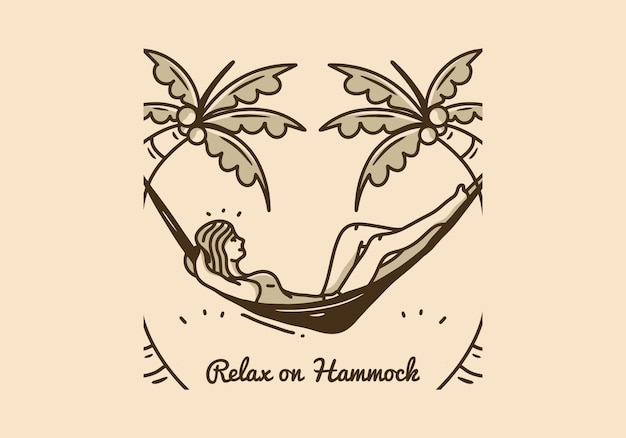This illustration presents a relaxed scene featuring a young woman lounging in a hammock, styled as a detailed cartoon sketch set against a tan, off-white background. The hammock, depicted in dark tones, stretches between two curved coconut palm trees. These trees arch inward due to the weight of the woman, creating a heart shape with their bending forms and lush leaves. The woman, who might be blonde, lies comfortably on the hammock, wearing a one-piece bathing suit with her arms resting behind her head and her legs extended. Surrounding the main image are stylized coconut motifs and intersecting line patterns, adding to the artistic design. Beneath the scene, the phrase "relax on a hammock" is inscribed, enhancing the laid-back ambiance of the illustration.